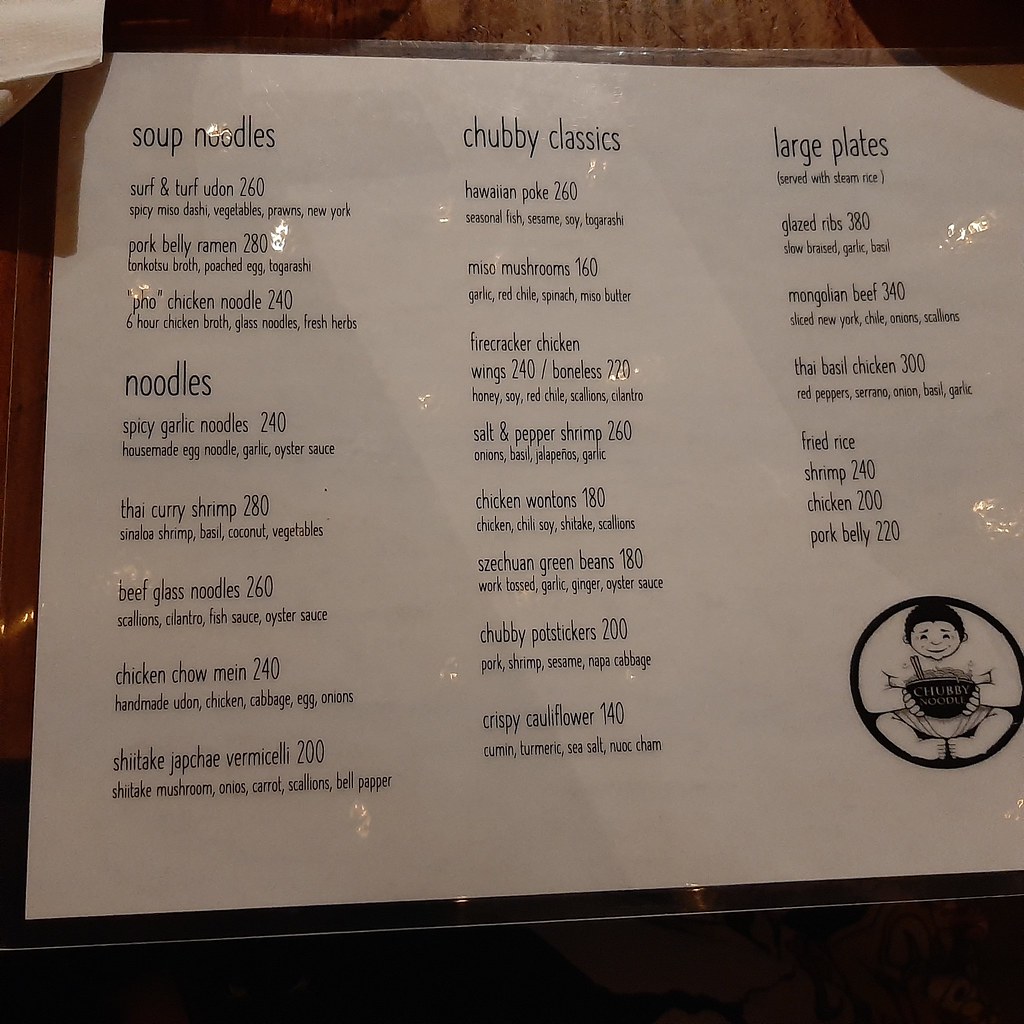The image showcases a detailed menu from Chubby Noodles, an Asian restaurant. At the top of the menu, sections are clearly labeled: Soup Noodles, Noodles, Chubby Classics, and Large Plates. 

Under **Soup Noodles**, the offerings include:
- **Surf and Turf Udon**
- **Pork Belly Ramen**
- **Uho Chicken Noodle**

The **Noodles** section lists:
- **Spicy Garlic Noodles**
- **Thai Curry Shrimp**
- **Beef Glass Noodles**
- **Chicken Chow Mein**
- **Shiitake Japchae Vermicelli**

In the **Chubby Classics** category, you can find:
- **Hawaiian Poke**
- **Miso Mushrooms**
- **Firecracker Chicken**
- **Salt and Pepper Shrimp**
- **Chicken Wontons**
- **Szechuan Green Beans**
- **Chubby Potstickers**
- **Crispy Cauliflower**

For **Large Plates**, the options are:
- **Glazed Ribs**
- **Mongolian Beef**
- **Thai Basil Chicken**
- **Fried Rice**
- **Shrimp**
- **Chicken**
- **Pork Belly**

Each menu item is accompanied by a brief description detailing the ingredients and preparation style, with prices listed adjacent to each dish.

In the bottom right-hand corner, there is a charming black-and-white drawing of a chubby Asian man. The restaurant's name, “Chubby Noodles,” is prominently displayed on a bowl within the illustration.